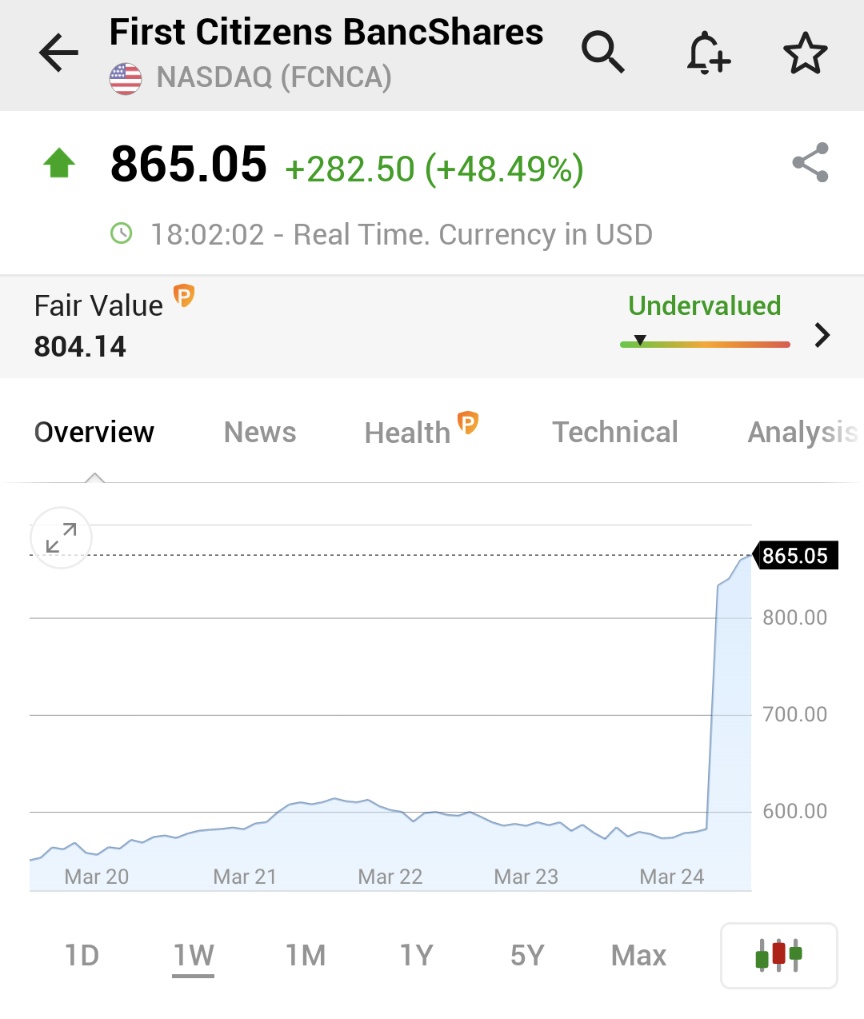This screenshot, taken from an individual's investment account, shows detailed performance metrics for their shares in First Citizens Bank Shares (NASDAQ: FCNCA). The share price has surged by an impressive 48.49%, resulting in an increase in the shares' value by approximately $282. Notably, the current fair value suggests that the shares remain relatively undervalued despite this upward trend. The price surge is recorded in real-time at 6:02 PM and is displayed in US dollars. The time frame for this significant price increase is within one week, although there are selectable options to view performance over one month, one year, and five years. As of the latest update, the shares are priced at $865.05 each.